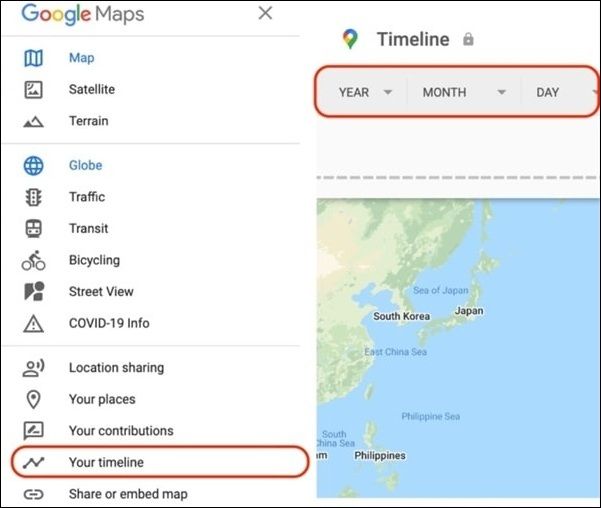The image depicts a detailed interface of a map-related application, presumably Google Maps. The interface is framed by a black outlined square and features the word "Google" in its characteristic multicolored text, followed by "Maps" in black, along with a small "X" symbol. Below this is a thin gray line separating the header from the main content.

The main section is divided into several categories and icons:

1. **Map Modes:**
   - **Map:** Represented by an icon of folded paper in blue next to the word "Map."
   - **Satellite:** Illustrated with a gray square containing various elements, denoted by the word "Satellite."
   - **Terrain:** Indicated by two triangles side by side, one filled and the other outlined and taller, next to the word "Terrain."
   - **Globe:** Shown by a blue globe icon beside the word "Globe" in blue.

2. **Layer Options:**
   - **Traffic:** Depicted with a traffic light icon and the text "Traffic."
   - **Transit:** Illustrated by a bus icon and the word "Transit."
   - **Bicycling:** Represented by a cyclist icon alongside "Bicycling."
   - **Street View:** Shown by an ambiguous icon with a circle, a square, and a partial triangle, followed by "Street View."
   - **COVID-19 Info:** Identified with an upward-pointing triangle, containing an unidentifiable element, next to "COVID-19 Info."
   - **Location Sharing:** Depicted by a person icon with two curved lines on the right and the phrase "Location Sharing."

3. **User Controls:**
   - **Your Places:** Shown with a typical map location pin icon and the text "Your Places."
   - **Your Contributions:** Indicated by a speech bubble with two gray lines, followed by "Your Contributions," with an orange outline.
   - **Your Timeline:** Represented by a zigzag line and the words "Your Timeline."
   - **Share or Embed Map:** Illustrated with a chain link icon and the phrase "Share or Embed Map."

4. **Timeline Interface:**
   - At the top right, there is another map symbol in different colors beside the word "Timeline" and a lock icon.
   - Below it, a rectangle with curved corners, outlined in orange and gray, shows date options labeled "Year," "Month," "Day," each followed by an arrow pointing down.

The bottom of the interface contains text that is too small to read clearly, and the background includes a visible map.